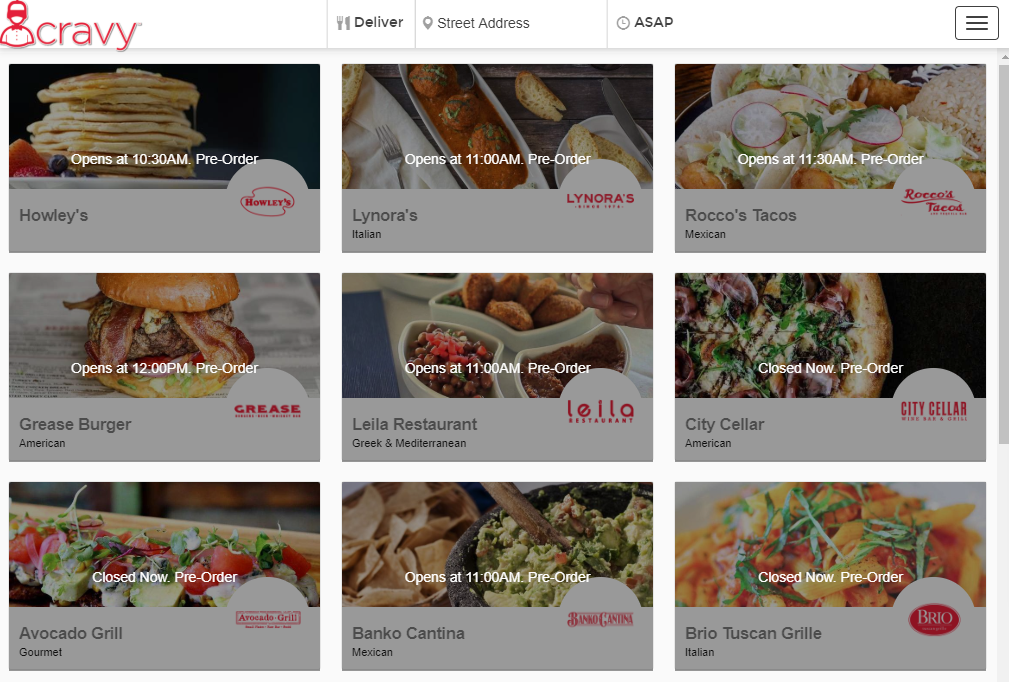A detailed image caption could be:

The image features a green foreground with a gray and white background, populated by numerous squares and rectangles. Centrally, there is a picture of either a chef or a man labeled "Cravey." The image also includes various icons such as a fork and knife, a street address marker, and a clock with the label "ASAP," along with a hamburger icon in a square.

The specifics of the content within these squares are as follows:
- "Howley's" - Opens at 10:30 AM (pre-order available)
- "Lenore’s Italian" - Opens at 11:00 AM (pre-order available)
- "Rocco's Tacos (Mexican)" - Opens at 11:30 AM (pre-order available)
- "Greaseburger (American)" - Opens at 12:00 PM (pre-order available)
- "Lila Restaurant (Greek Mediterranean)" - Opens at 11:00 AM (pre-order available)
- "City Cellar (American)" - Currently closed (pre-order available)
- "Avocado Grill (Gourmet)" - Currently closed (pre-order available)
- "Banco Cantina (Mexican)" - Opens at 11:00 AM (pre-order available)
- "Brio Tuscan Grill (Italian)" - Currently closed (pre-order available)

On the right side of the image, there is a gray scroll bar, indicating that there are more options or details beyond the current view.